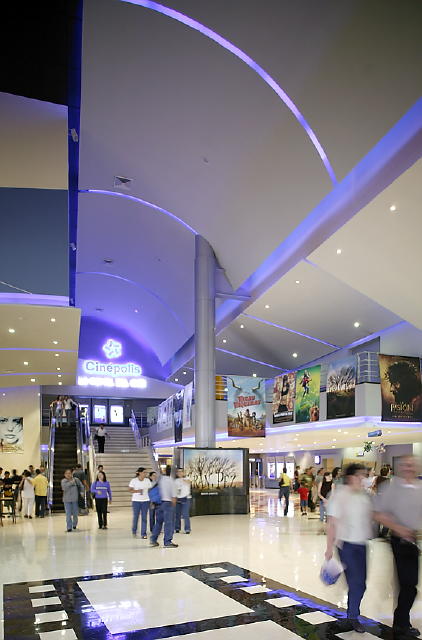The image captures an expansive indoor space that appears to be part of a shopping mall or a cinema complex. The ground floor features a distinctive multicolored tile flooring in a pattern that mimics a filmstrip, with reflective white tiles and a black path down the center leading to a prominent white staircase. At the top of the staircase, a neon sign glows with the text "Cinepolis," partially legible as "C-I-N-E-P-O-L-I-S," though some additional letters are out of focus.

The scene is bustling with activity, as various people walk around, mostly out of focus but concentrated near the central staircase. On the right side of the image, there are storefronts and several movie posters, including those for "Passion of the Christ," "Big Fish," and "Honey" featuring Jessica Alba. The walls of the establishment are beige, adorned with recessed lighting that highlights the high, curved ceiling supported by a giant metal pole.

Overall, the setting is well-lit and clearly indoors, likely within a shopping mall that includes a cinema. The environment combines commercial and entertainment elements, with a tiled floor, prominent signage, and bustling foot traffic to create a lively atmosphere.